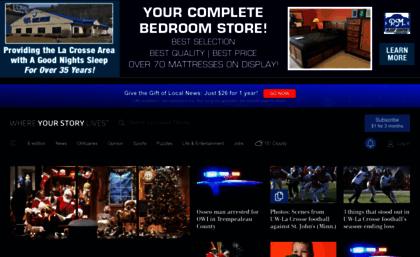A captured image of a website banner prominently features the word "Tribune" in large letters at the top. The main image on the left side of the banner portrays a judge's gavel placed before a set of law books, accompanied by the headline: "New Judge Chosen for Todd Gieck Case in Trempealeau County." The name "Todd Gieck" (spelled G-I-E-C-K) and "Trempealeau County" (spelled T-R-E-M-P-E-A-L-E-A-U) are detailed in the text. Below the headline, there are six smaller images, each corresponding to different articles, though their text is too small to decipher. These smaller images include: another picture of a gavel, a group of people smiling at the camera, a photo depicting a road or possibly a railroad crossing, a person standing alone, a scene of individuals outdoors, and another outdoor shot featuring people amidst buildings.